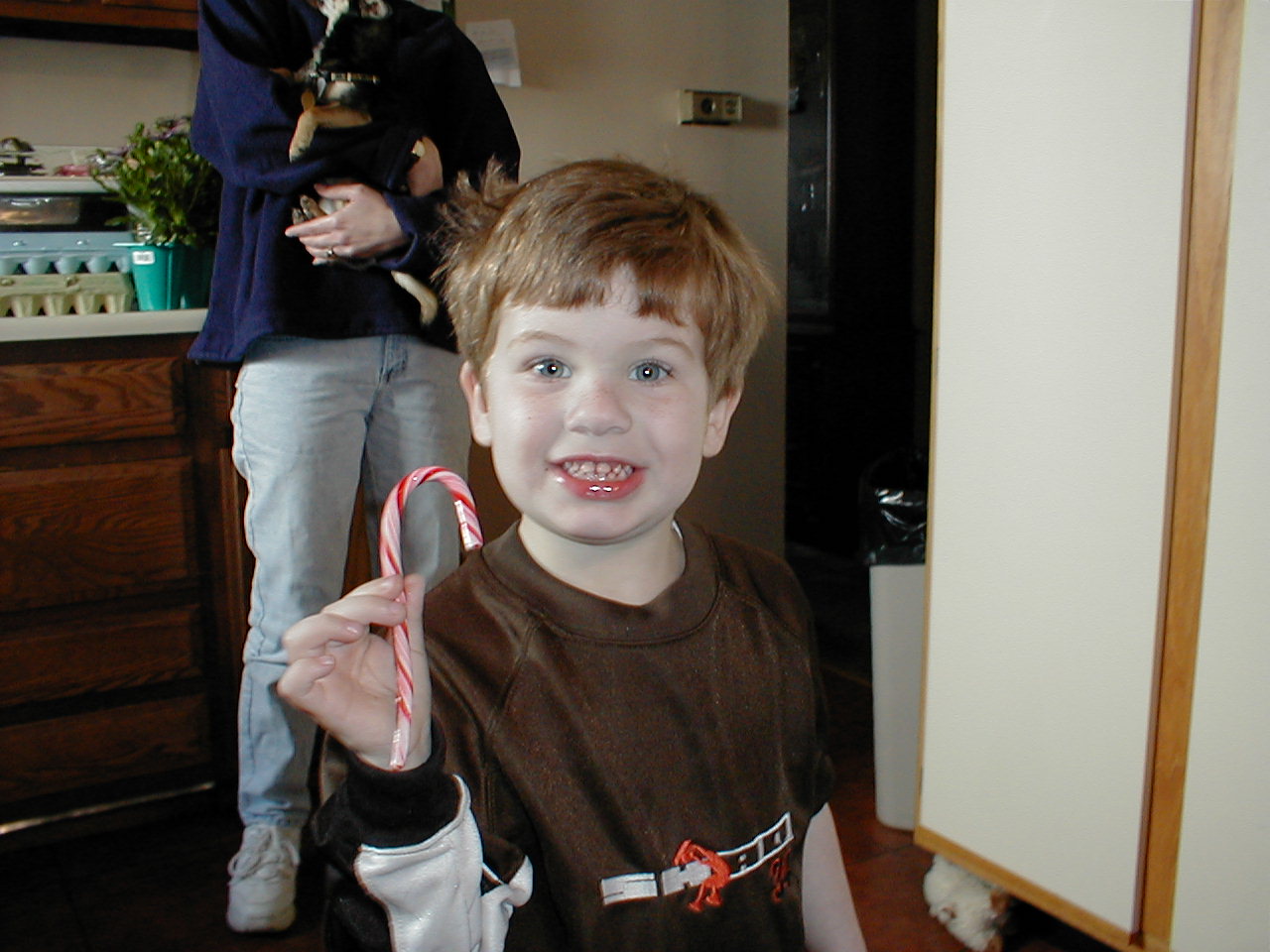In the photograph, a young boy, approximately 5 or 6 years old, is standing indoors, possibly in a kitchen, holding up a full-sized red and white candy cane in his right hand. The boy, who is very pale with hair that appears to be a reddish-brown or light brown, is smiling directly at the camera. He is wearing a long-sleeved brown shirt featuring the name "Shaq," referring to Shaquille O'Neal. Behind the boy, there is a man visible from the neck down, dressed in a dark blue sweater, light blue jeans, and white sneakers. The man appears to be holding a small, wriggly black dog, which has a collar. The setting includes wooden cabinets, countertops, a few egg cartons, and various other kitchen items.